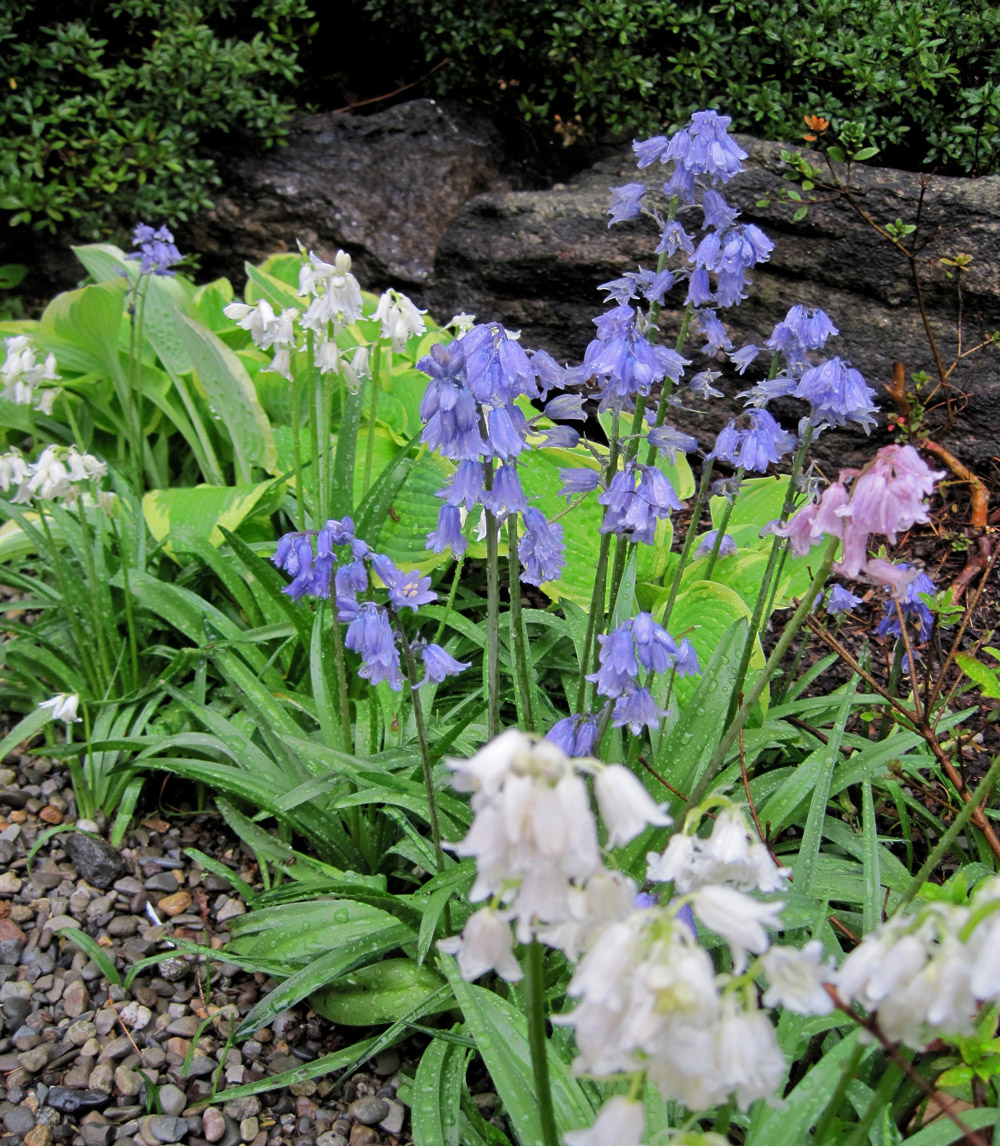In this close-up outdoor photograph, vibrant shades of nature are vividly captured in a well-maintained garden. The forefront of the image showcases clusters of upside-down, bell-shaped flowers in brilliant hues of purple, interspersed with patches of white and softer pink varieties. These flowers, identified as bluebells, exhibit long, slender green leaves, contributing to the lush green foliage that frames the scene. Surrounding the garden bed is a mix of small stones, pebbles, and gravel that add texture and contrast to the colorful display.

Behind the flowers, there are large gray stone formations creating a sturdy backdrop, further accentuated by the presence of some gray gravel at the base. Just behind these stones are very dark green bushes or hedges, with an occasional glimpse of orange flowers peeking through, adding another layer of color. The background is completed with hints of additional greenery, possibly from hostas or other garden plants, and some branches lying on the ground. This photograph captures the beauty and meticulous care of the garden, highlighted by the interplay of colors and natural elements.